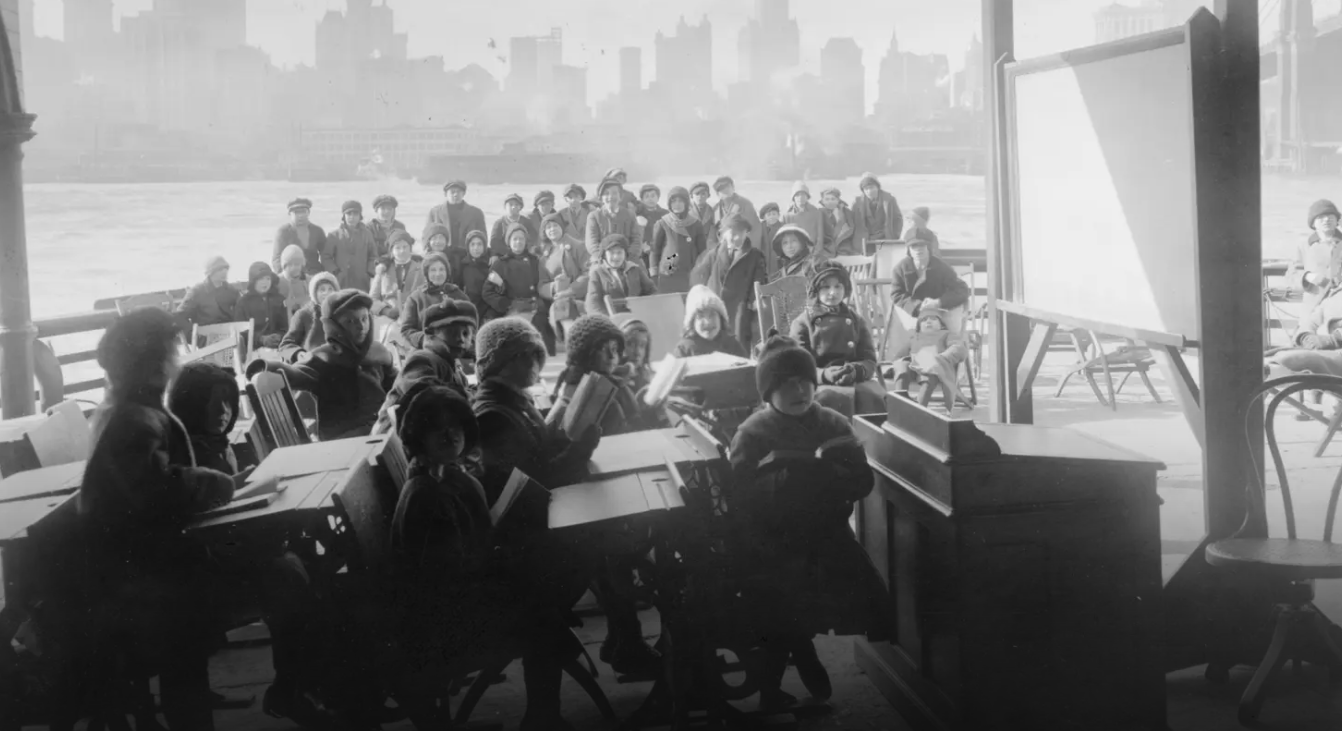This black and white vintage photograph captures an intriguing outdoor scene that seems to depict a makeshift classroom set against an urban skyline. The cityscape in the far background is dominated by tall, light gray buildings, possibly New York, under an overcast sky. Just in front of the skyline, a large waterway adds depth to the image. 

Closer to the foreground, rows of children are seated at very old-fashioned desks, each wearing knitted hats and heavy coats, suggesting a chilly day. Their youthful faces and attire, which appears outdated by modern standards, make it clear they are schoolchildren from a bygone era. A pulpit and an old-fashioned chair stand in front of the desks, accompanied by a board likely used for their lessons.

Behind the children, a crowd of adults also dressed in hats and coats look on with expressions that suggest a mix of expectancy and hope. Wooden chairs are scattered among them, indicating some are seated while others stand, all gazing toward the camera. The photograph, entirely monochromatic with shades of gray, black, and white, encapsulates a moment in time where education and urban life meet against a wintry urban backdrop.